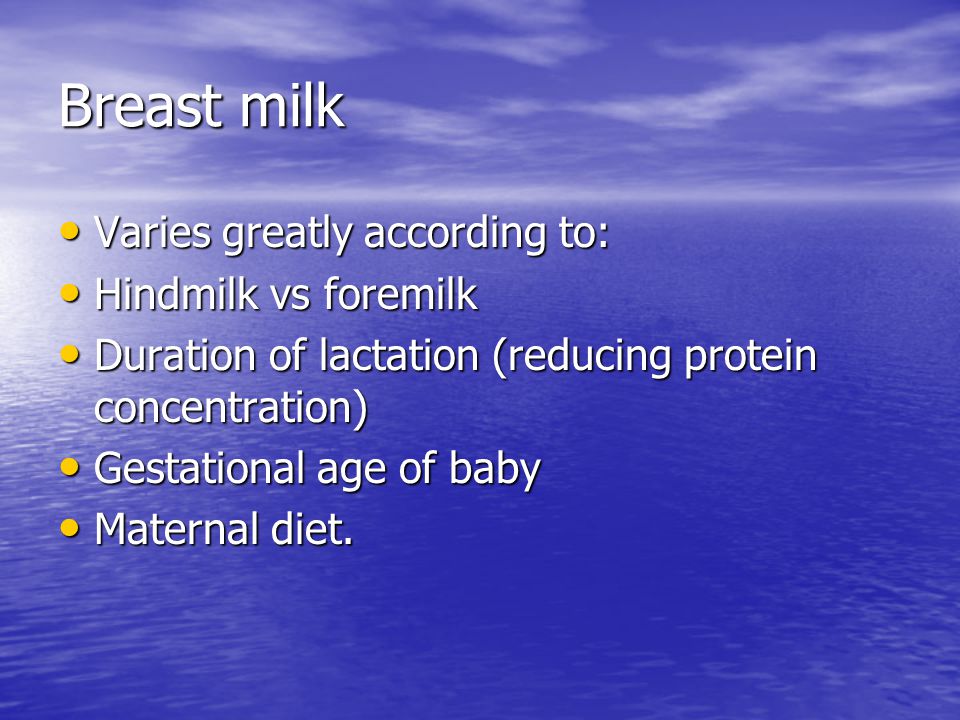The image is a slide from a PowerPoint presentation with a background featuring an edited photo of the ocean and sky, tinted blue for visual appeal. The sky occupies the top quarter of the image, with the ocean filling the rest. The slide is centered around the title "Breast Milk," written in large white text with a dark shadow background, positioned in the upper left corner. Below the title, a series of yellow bullet points in slightly smaller white text provide detailed information about breast milk. The bullet points highlight various factors, including how breast milk varies greatly according to hind milk versus foremilk, the duration of lactation, the reducing protein concentration, the gestational age of the baby, and the maternal diet. This detailed and visually engaging slide serves as an educational tool on breast milk.